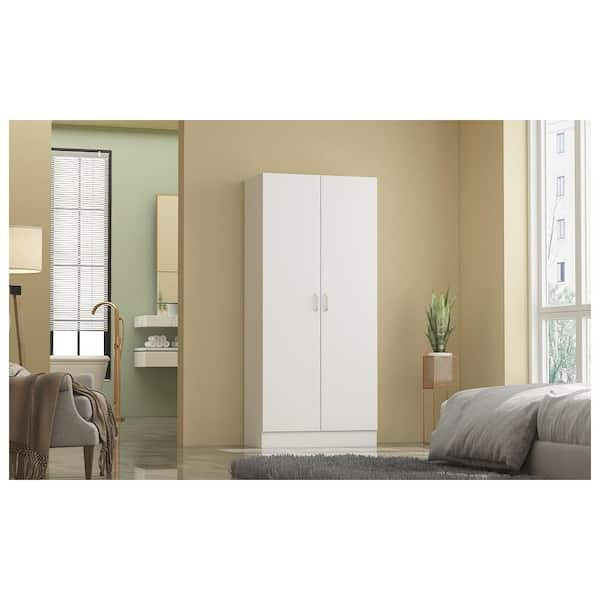This photograph captures a cozy den with detailed decor and furnishings. At the center is a tall, white cabinet with two doors, set against a brownish, beige wall. To the right, nestled in the corner, is a green potted plant that stands approximately 12 to 14 inches tall. The left side of the image reveals a chair draped with an Afghani shawl or blanket, beside which stands a lit lamp with a white lampshade. The den leads into another room, possibly a kitchen or bedroom, featuring a green wall and a window with multiple panes. Visible through a large window in this adjoining room, you can glimpse some greenery and a neighboring multi-story building. Additionally, a beige sofa or bed can be seen, complemented by a plush, full gray rug. The scene is completed with various thoughtful details, such as a cane in front of the chair and additional cabinets or storage elements in the background, contributing to the room's warm and inviting atmosphere.